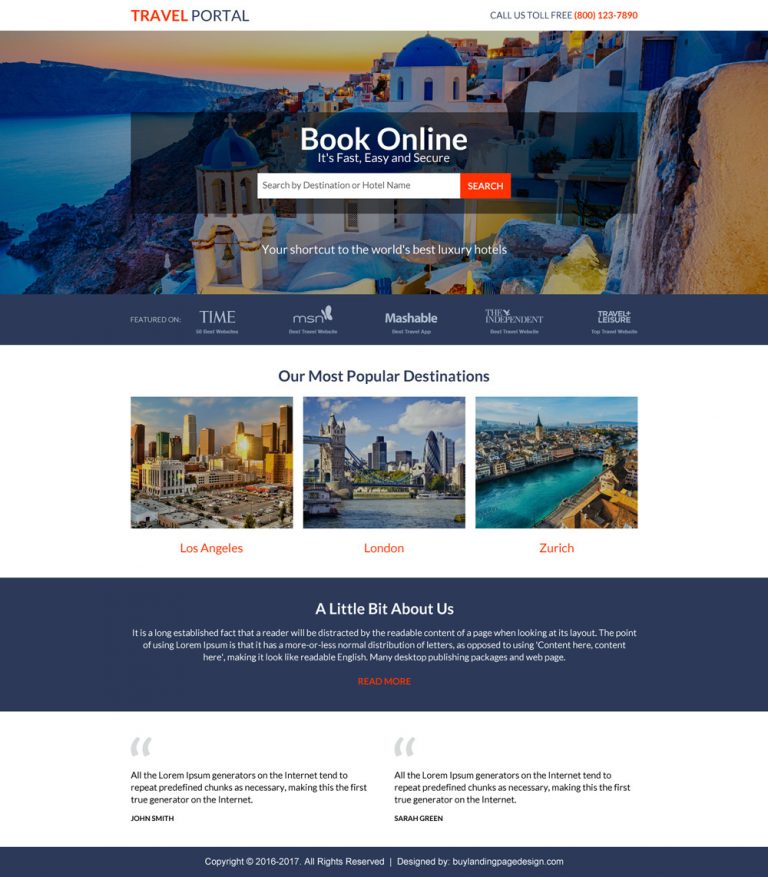**Detailed Descriptive Caption:**

The image portrays a vibrant travel website with a predominantly white background accented by bright orange, white, and medium royal blue elements, creating a lively and inviting aesthetic. At the top of the page, "Travel Portal" is prominently displayed in stylish orange and black text. Opposite this, to the right, there is contact information in black and orange text that reads, "Call Us Toll-Free [800-123-7890]".

A large, captivating image of a sunset graces the center of the webpage. The sunset showcases a splendid palette of white, orange, pink, and light blue hues. The scene includes a rocky region at the forefront and a serene body of blue water, with tightly packed white stone buildings featuring dark blue arched rooftops adorned with crosses on the right.

Superimposed on the sunset is a sheer black rectangular box with white text proclaiming, "Book Online. It's fast, easy, and secure." Below this message is a user-friendly white search bar marked by light gray placeholder text, "Search by Destination or Hotel Name", and a bright orange search button that says "Search".

An inspiring headline in white text, "Your Shortcut to the World's Best Luxury Hotels", is positioned below. This section is complemented by a solid dark blue border at the bottom, displaying white text and logos from five reputable platforms: Time Magazine, MSN, Mashable, The Independent, and Travel Plus Leisure, signifying the website's prominence.

Continuing downward, the section titled "Our Most Popular Destinations" is presented in dark blue text against a white background. It features three eye-catching square images labeled "Los Angeles", "London", and "Zurich" in orange text. These images capture bright blue skies, white puffy clouds, city skylines, and expansive blue waters.

Following this, a dark blue rectangular box with white center text titled "A Little Bit About Us" contains placeholder text, explaining the use of Lorem Ipsum for designers. Below this is a bold orange link labeled "Read More".

The site further includes inspirational quotes in light blue stylized quotation marks. One quote reads, "All the Lorem Ipsum generators on the Internet tend to repeat predefined chunks as necessary, making this the first true generator on the Internet," credited to John Smith. Another similar quote is attributed to Sarah Green.

The footer of the page features a dark blue border spanning its width, with white text displaying the copyright notice, "© 2016-2017. All rights reserved. Designed by ByLandingPageDesign.com".